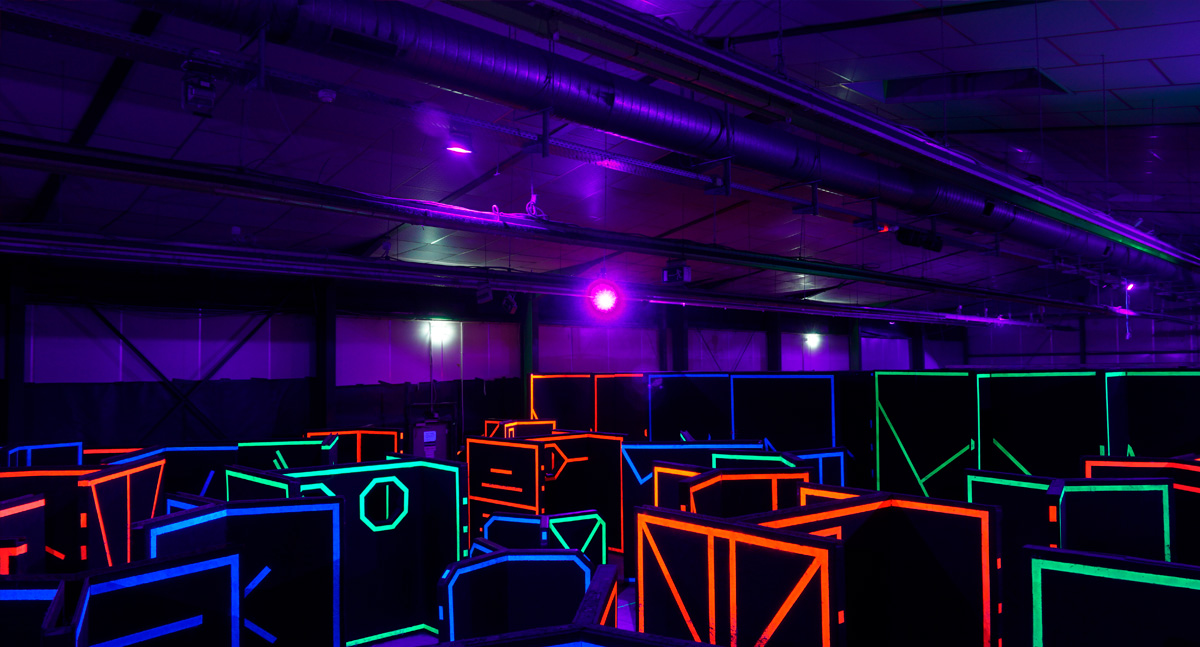The image depicts a dimly lit interior space, possibly a warehouse or play building, with a vast metal frame structure and a drop ceiling adorned with exposed ductwork and fluorescent lighting. The room is filled with black furniture, including square desks, chairs, and partitions, some resembling study carousels. These objects are strikingly illuminated in vibrant neon colors—red, blue, fluorescent green, orange, and yellow—that create a glowing outline against the dark backdrop, reminiscent of a laser tag arena or a storage area for club furnishings. The ceiling reveals heating and cooling tubes and steel beams supporting the structure, while the absence of windows adds to the enclosed and surreal atmosphere.